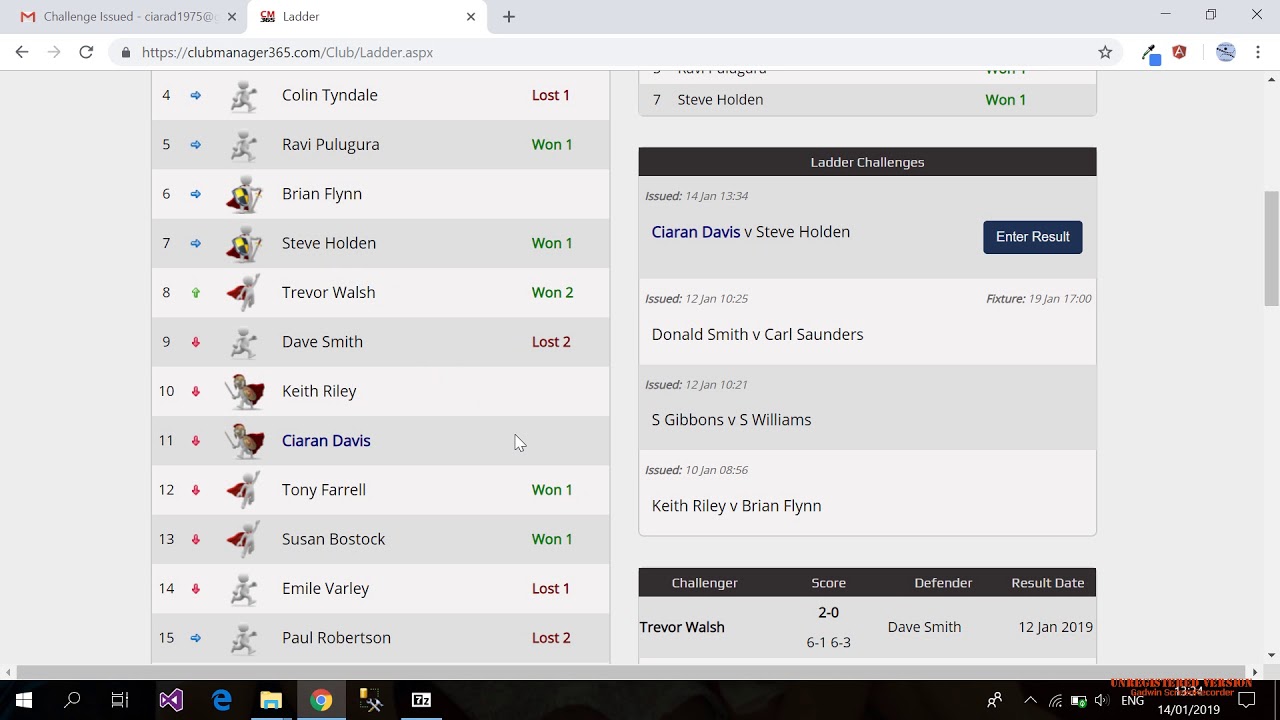This image is a detailed screenshot of a computer screen displaying a specific interface, possibly related to a sports or gaming club management system accessed via clubmanager365.com. 

At the top left corner, two browser tabs are visible; the first is labeled "Challenge," and the second, though partially obscured, seems to be associated with an email platform. On the right-hand side of the browser, the word "Ladder" is displayed prominently. Just below, the URL "clubmanager365.com" is clearly visible.

Further down on the right, there are three identifiable icons followed by a vertical ellipsis (three vertical dots). Adjacent to these is a star icon located at the end of the search bar.

On the left side of the screen, a list of individuals is presented in a vertical column, with numbers ranging sequentially from 4 to 15. Next to each number is a corresponding name, followed by match results noted in either red (for losses) or green (for wins). The pattern of results reads: lost, won, 11, 11, 12, lost 2, 11, 11, lost 1, lost 2.

Notably, to the right, the entries for number 7, Steven Holden, display an 11, and the words "Ladder Challenges." Further below, the name Claire Davis is listed involving a challenge to Steve Holden, with a mention of results and three additional matchups. Subsequently, another challenge by Trevor Walsh reveals the score, defender, and result.

Towards the bottom of the screenshot, a series of nine computer icons is arranged. Additionally, there are several more icons visible to the right side, concluding the displayed content of this interface.